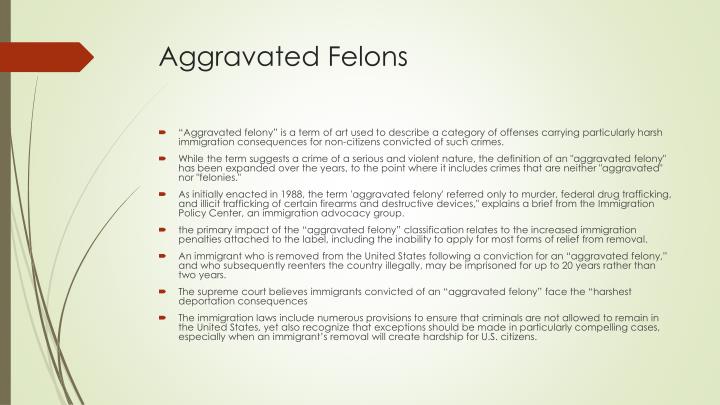The image depicts an informative slide from a PowerPoint presentation, titled "Aggravated Felons," highlighting the serious deportation consequences faced by immigrants convicted of such crimes. The slide is set against a light greenish background with a design featuring a small bush and a thin, brownish-colored border on the left. A prominent red arrow at the top points to the heading in large, black letters. Beneath the heading, there are seven red bullet points aligned vertically. Each point elaborates on how the term "aggravated felony," originally defined in 1988 to include severe offenses like murder, federal drug trafficking, and illicit firearms trafficking, has been broadened over the years to encompass crimes that are neither aggravated nor felonies. The slide emphasizes the harsh immigration penalties associated with this classification, such as the ineligibility for most forms of relief from removal and potential imprisonment of up to 20 years for re-entering the US illegally post-deportation. The Supreme Court is specifically noted for its stance that immigrants convicted of aggravated felonies endure the most severe deportation ramifications. The information is derived from a brief by the Immigration Policy Center and an Immigration Advocacy Group, suggesting the slide's alignment with pro-immigrant support viewpoints.